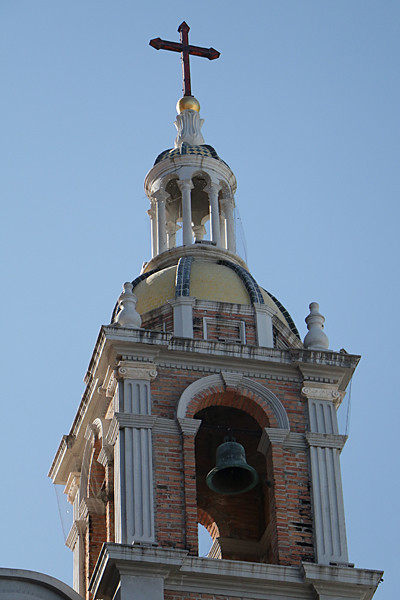This vertically aligned, upward-angled photograph captures the upper section of a chapel or church against a solid blue sky, illuminated by sunlight. The centerpiece is a bell tower, primarily constructed of brick and accented with white stone, particularly in the engraved pillars and archways at the corners. The bell itself is a static, dark gray metal, hanging within the arched opening, with visibility through the arch revealing similar openings on other sides. The structure progresses upwards to a smooth, rounded dome adorned with black markings, transitioning into another open area bordered by white pillars, contributing to a cathedral-like appearance. At the peak, a dark cross sits atop a gold ball, completing the intricate and majestic look of this ecclesiastical architecture.